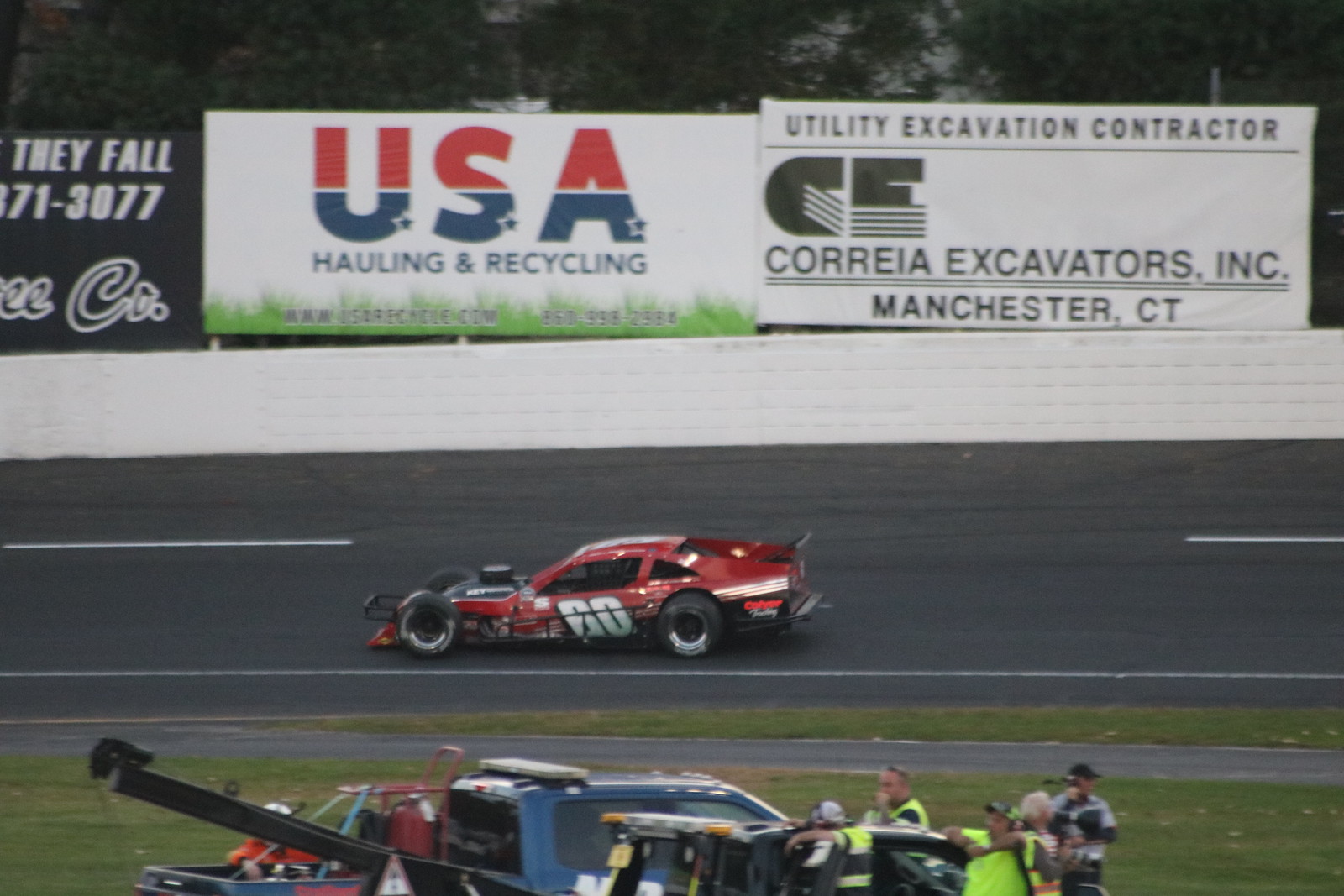This color photograph depicts a dynamic daytime scene at a racetrack. At the center of the image, a red racecar bearing the number 60 (or 6060) with white stripes and a black bumper is prominently featured with its hood popped, revealing the engine. This car is positioned on the track, possibly moving towards the left side of the image. In the foreground, three men wearing high-visibility vests stand next to three tow trucks parked on the grassy area adjacent to the track. The background features a series of advertising billboards on the guardrail, including one for USA Hauling and Recycling and another for Corelia Excavators Incorporated, a utility excavation contractor based in Manchester, Connecticut. The image captures a moment rich in detail and activity, with the racecar and tow trucks evoking the high-energy atmosphere typical of a racetrack setting.